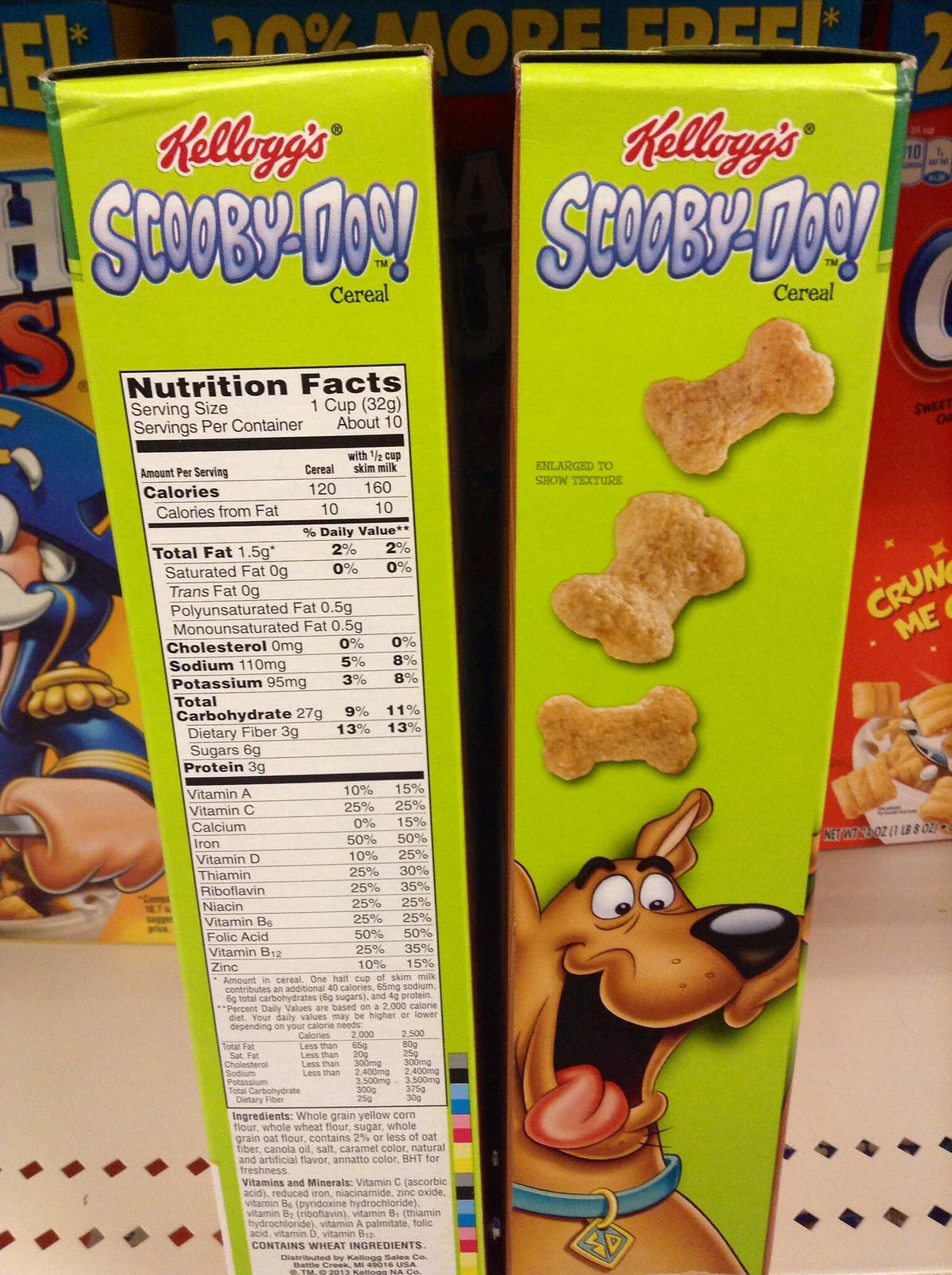This image features two Kellogg's Scooby-Doo cereal boxes positioned side by side, emphasizing the left and right sides of the boxes rather than the front or back. The left box displays the nutritional facts panel, detailing information like serving size, which is one cup, along with other nutritional data. The right box showcases the branded side with a vibrant image of Scooby-Doo, accompanied by three of the cereal pieces, likely representing the shapes and colors found inside. The setting appears to be a grocery store aisle, evidenced by the visible shelving and an assortment of other cereal brands, including Captain Crunch, in the background.